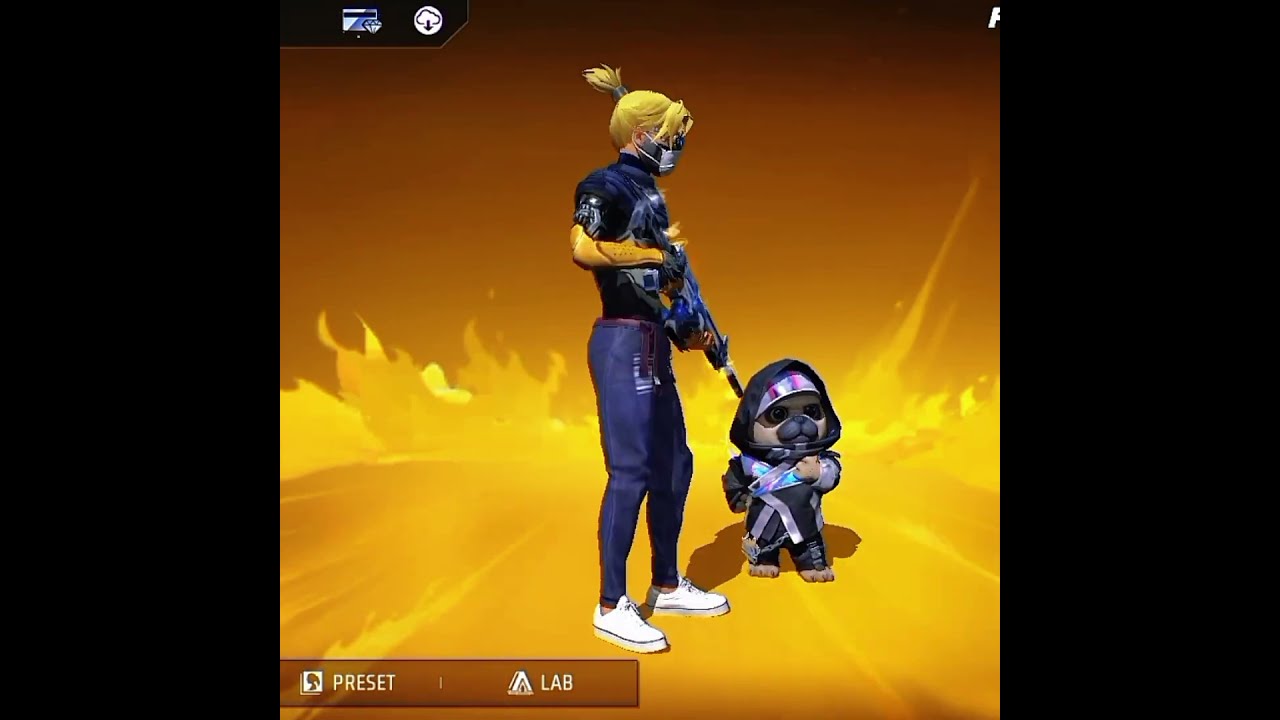The image is a vibrant and intense screenshot from a video game featuring two central characters standing against a backdrop of flames. At the center, a blonde woman with her hair pulled up into a bun and white bangs cascading over her face, dons a white face mask. She is dressed in a layered outfit that includes a purple and black shirt, a blue shirt, and yellow arm coverings. She is also wearing blue pants and white tennis shoes. The woman is firmly gripping a large assault rifle with both hands, one hand under the butt and the other under the center stock, pointed downwards towards the second character.

Beside her stands an anthropomorphized pug in a black ninja gi, adorned with ribbons in purple, white, and pink colors. The pug is in a combat-ready stance with its fists raised, its black muzzle and shadowed eyes contributing to its formidable appearance. The characters are positioned on a yellow surface that transitions into bright, engulfing flames at the bottom of the scene. The left side of the image features text labels that read "Preset" and "Lab," while the upper left corner contains a white circle with a cloud emblem and a down arrow next to another icon resembling a credit card with a diamond on it.